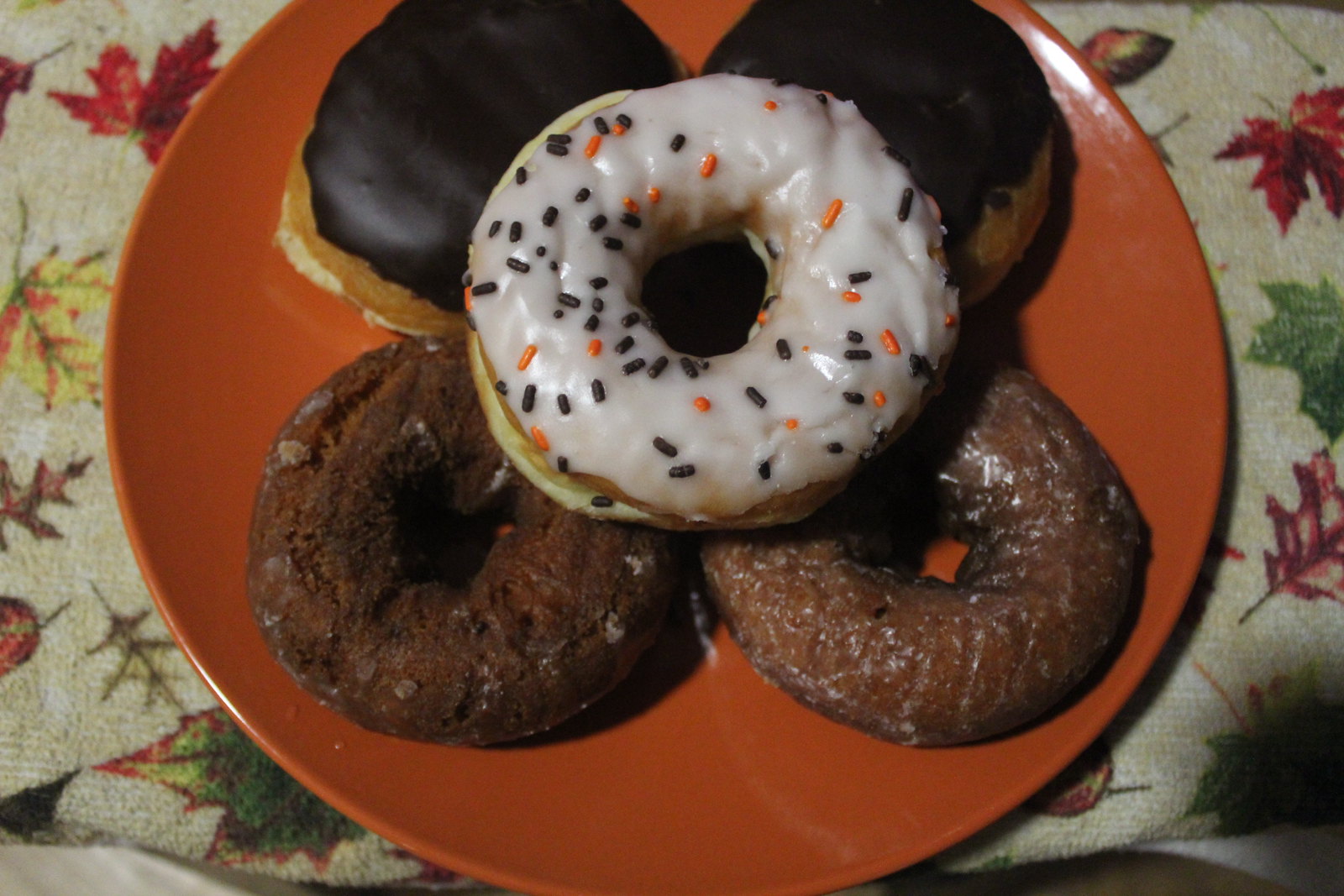On a table adorned with a beige tablecloth featuring vibrant red, green, and yellow autumn leaves, sits a striking orange plate arranged with five decadent doughnuts. At the center of the arrangement, a prominent doughnut with white glaze is generously sprinkled with festive black and orange Halloween sprinkles. Flanking this centerpiece, at the top, are two chocolate-covered doughnuts, each with a rich, glossy chocolate frosting accent. Below, on the left side, lie two classic Boston cream doughnuts, their smooth chocolate glaze hiding a creamy surprise within. Completing the array on the right are two pumpkin-flavored cake doughnuts, one plain and one slightly glazed, embodying the essence of the autumn season. This tempting collection captures the cozy and festive spirit of Halloween and fall in one delicious display.